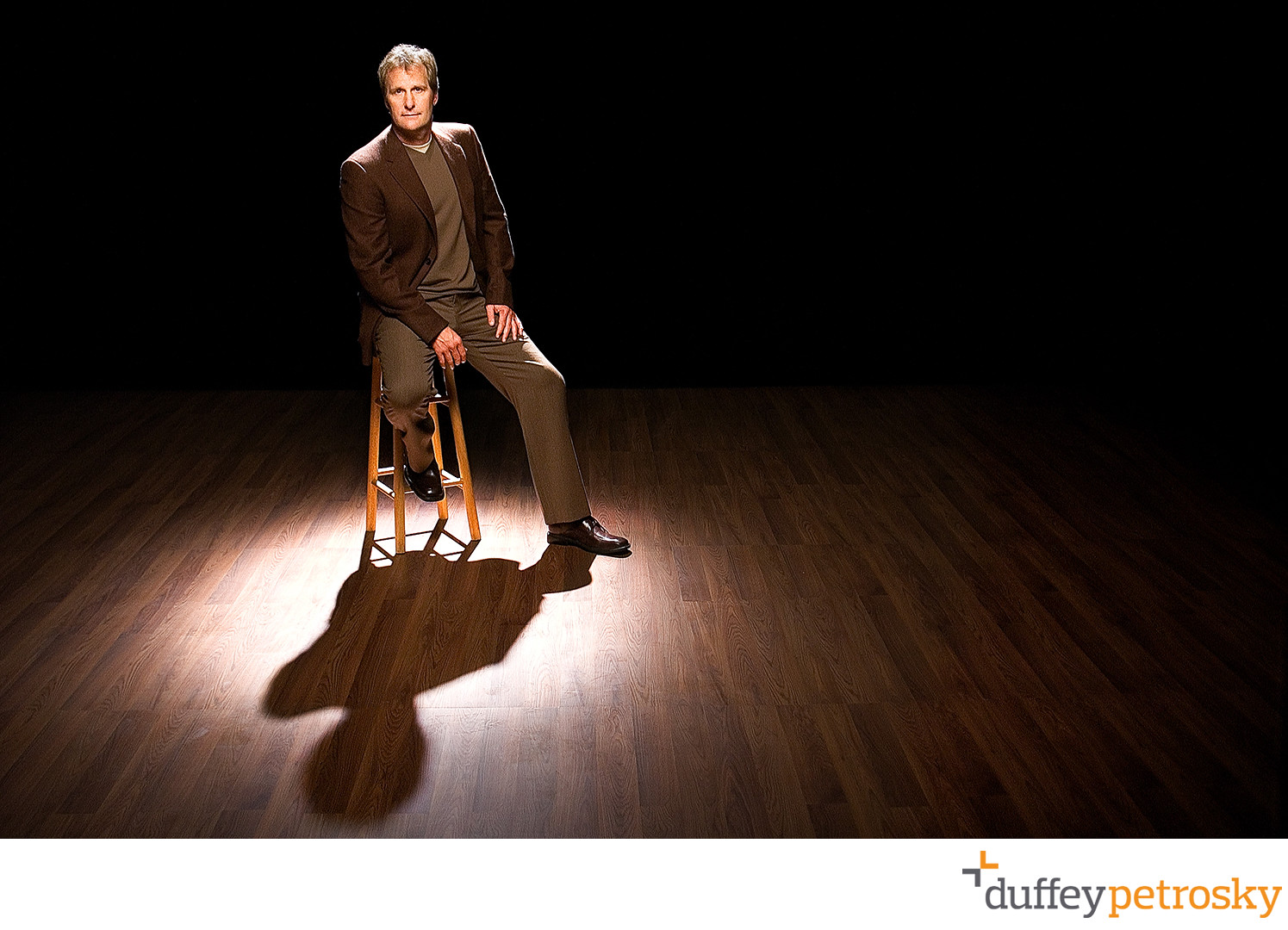The wide rectangular photograph centers on a man positioned in the top left corner, sitting on a light brown wooden stool that casts a stark shadow beneath it. The scene features a stage-like setting with a simplistic beauty; the backdrop is a pure, unbroken black, creating a striking contrast against the glossy dark brown wooden floor. The narrow planks of the floor stretch towards the horizon line, adding depth to the setting. The man, with blonde hair, gazes forward with a confident, almost challenging look. He wears grey pants, a greenish-grey sweater layered under a dark grey blazer, and has one leg bent with the heel resting on the stool ledge, while the other leg extends outward, bent at the knee. The spotlight illuminates him, emphasizing the darkness around and beneath the stool. The photo, credited to Duffy Petrovsky, captures an evocative, minimalist composition.